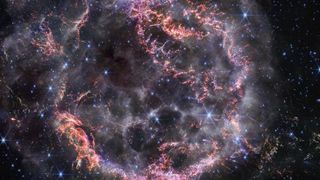This image appears to be a detailed photograph of a distant galaxy, possibly captured with a telescope. The background is a deep, dark black, showing a myriad of twinkling stars. The foreground features a striking burst of colors and forms, primarily composed of clouds and gas in shades of pink, purple, orange, and gray. These clouds and gases appear to swirl in a somewhat circular formation, reminiscent of a galaxy or nebula, against the star-studded backdrop. The overall composition gives the impression of a vibrant astronomical phenomenon, yet it's hard to pinpoint if the swirling colors are planetary surfaces, atmospheric clouds, or simply colorful celestial vapors. The image does not contain any text, creatures, or identifiable objects, making its exact context unclear.